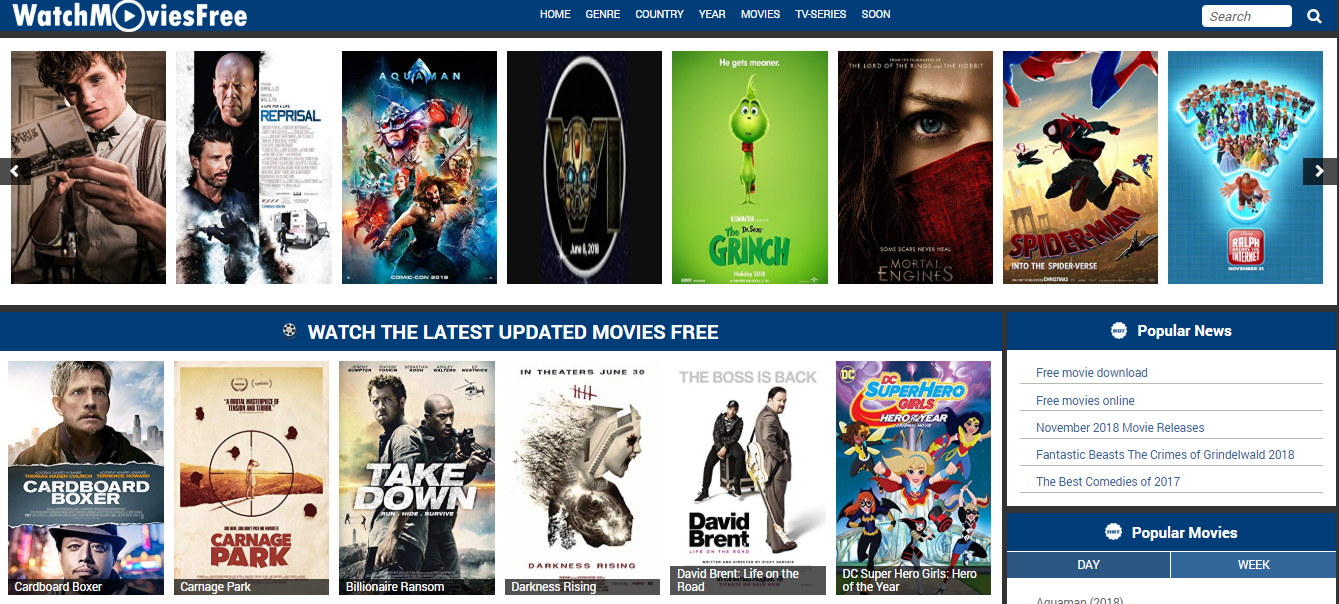Here's a detailed and cleaned-up version of the caption:

---

The image depicts the homepage of a website titled "Watch Movies Free," which features a predominantly blue background. At the top, a navigation bar lists several menu options in white capital letters: Home, Genre, Country, Year, Movies, TV Series, and Show. Adjacent to these options is a search bar.

Beneath the navigation bar, there is a row of eight movie covers as follows:
1. A movie featuring an actor in a bow tie and suspenders holding a pamphlet.
2. "Appraisal," possibly starring Bruce Willis.
3. An animated-looking film, possibly "Avatar."
4. A movie with a character wearing a black mask within a white circle.
5. The live-action version of “The Grinch That Stole Christmas.”
6. An actress with a red mask and a serious expression.
7. A "Spider-Man" movie.
8. An animated film featuring various characters.

Below this row is a caption that reads, "Watch the latest updated movies for free." Another row of movies is displayed, consisting of:
1. "Cardboard Boxer."
2. "Carriage Parts."
3. "Take Down" with Samuel L. Jackson.
4. An unidentified film featuring some Bates theme elements.
5. "David Brent."
6. An animated superhero film which may include Wonder Woman and other characters.

To the side is a menu box labeled "Popular News," with five entries advertising various movie-related news articles. These include headlines about movie releases, "Fantastic Beasts," "Best Comedies of 2017," along with links to popular movies and day/week viewing options.